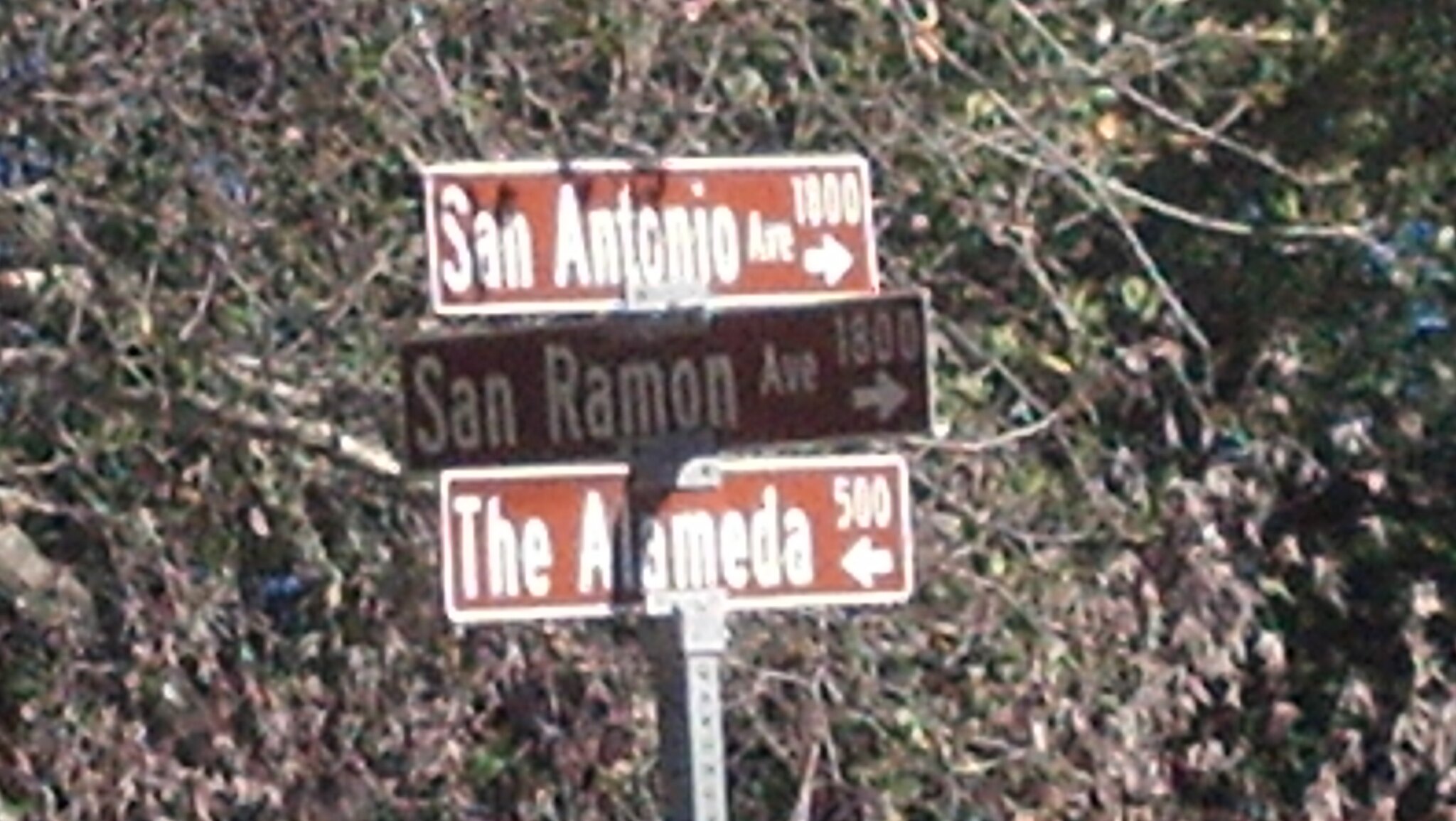This color photograph captures a trio of street signs stacked on a gray perforated metal pole, set against a backdrop of trees with a mix of dead and bright green leaves under a blue autumn sky. The top sign reads "San Antonio Ave, 1800," with an arrow pointing to the right. Below it, the sign says "San Ramon Ave, 1800," also with a right-pointing arrow. The bottom sign states "The Alameda, 500," featuring a left-pointing arrow. All three signs are a rusty brown hue with white lettering and trim. The photograph is taken from a somewhat close-up perspective, allowing clear visibility of the detailed metal structure and foliage around them.